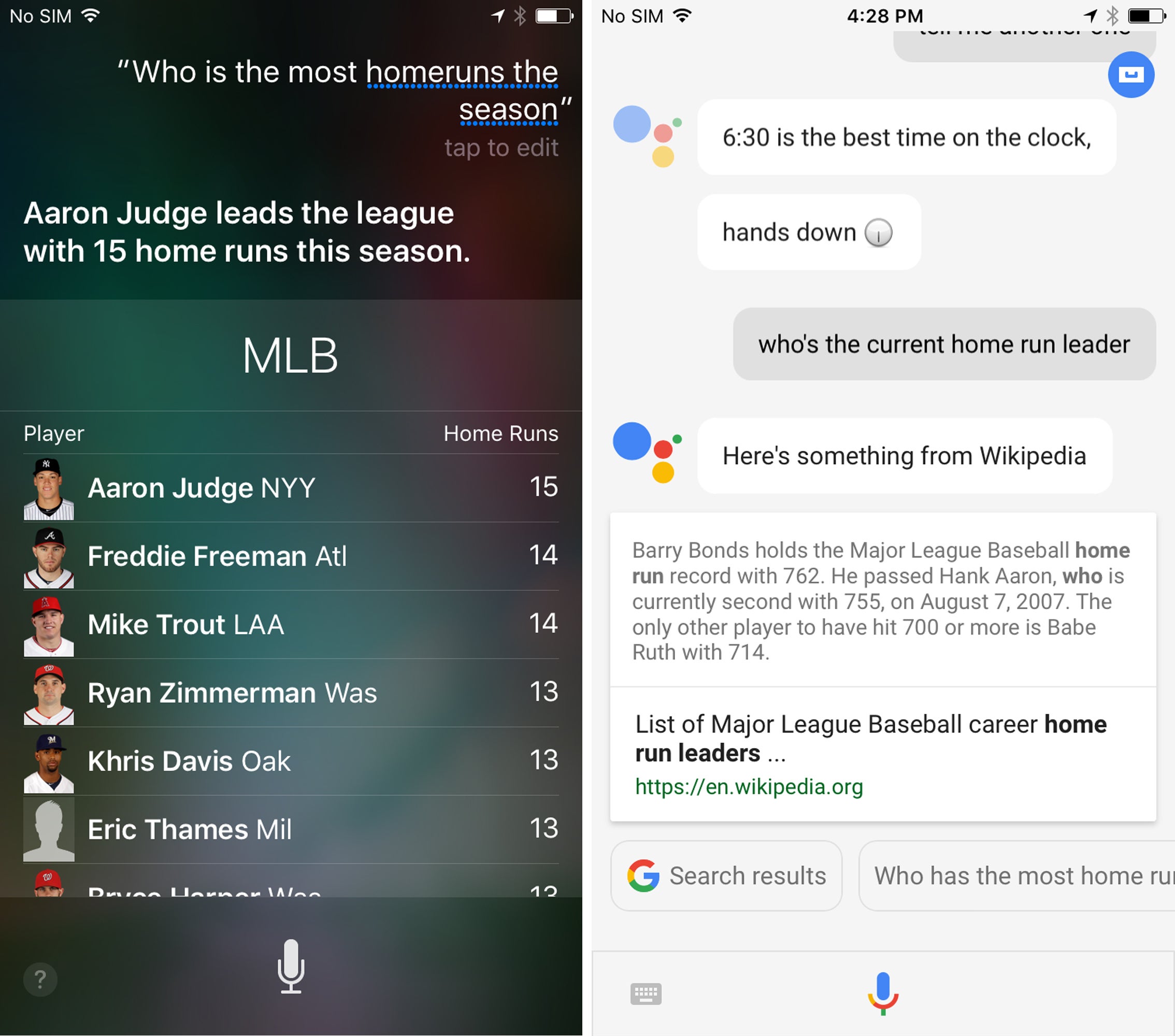The image, set against a solid white background, displays a screenshot from a cell phone. At the top of the screen, white text indicates "No SIM" along with a Wi-Fi icon and a half-full battery icon. Just below this, more white text poses the question, "Who is the most home runs this season?" with an option to "Tap to edit." The information reveals that Aaron Judge leads the league with 15 home runs this season.

Beneath this statement is a greenish box labeled "MLB," accompanied by a detailed player list on the left and their corresponding home run totals on the right:

1. Aaron Judge, NYY - 15 home runs
2. Freddie Freeman, Atlanta - 14 home runs
3. Mike Trout, LA - 14 home runs
4. Ryan Zimmerman - 13 home runs
5. Eric Mill - 13 home runs

On the right side of the image, there's a conversation thread. One message reads, "6:30 is the best time on the clock. Hands down." A response beneath it asks, "Who's the current home run leader?" 

The screenshot provides a snapshot of pertinent MLB statistics and a snippet of a casual conversation, all combined within a clean, minimalist layout.